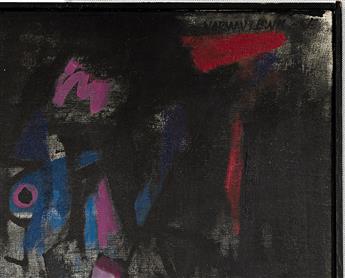The image is a compelling abstract painting that predominantly features dark colors, creating a moody and intense aesthetic. The canvas appears to be mainly black, possibly with layers of dark paint applied over a lighter background. Notably, there are various vibrant accents throughout. In the top right and near the center, striking red brushstrokes suggest an attempt to cover or obscure something. On the bottom left, there is a distinct eye-like shape, outlined in black with hues of blue, magenta, and black creating an illusion of an eye staring back at the viewer. Scattered across the painting are additional vibrant streaks of pink and blue, adding dynamic pops of color. Above the eye on the top left, an 'M' in pink appears inscribed, while just above the right red stroke, there's a barely legible black text that looks hand-drawn, contributing to the enigmatic quality of the piece.